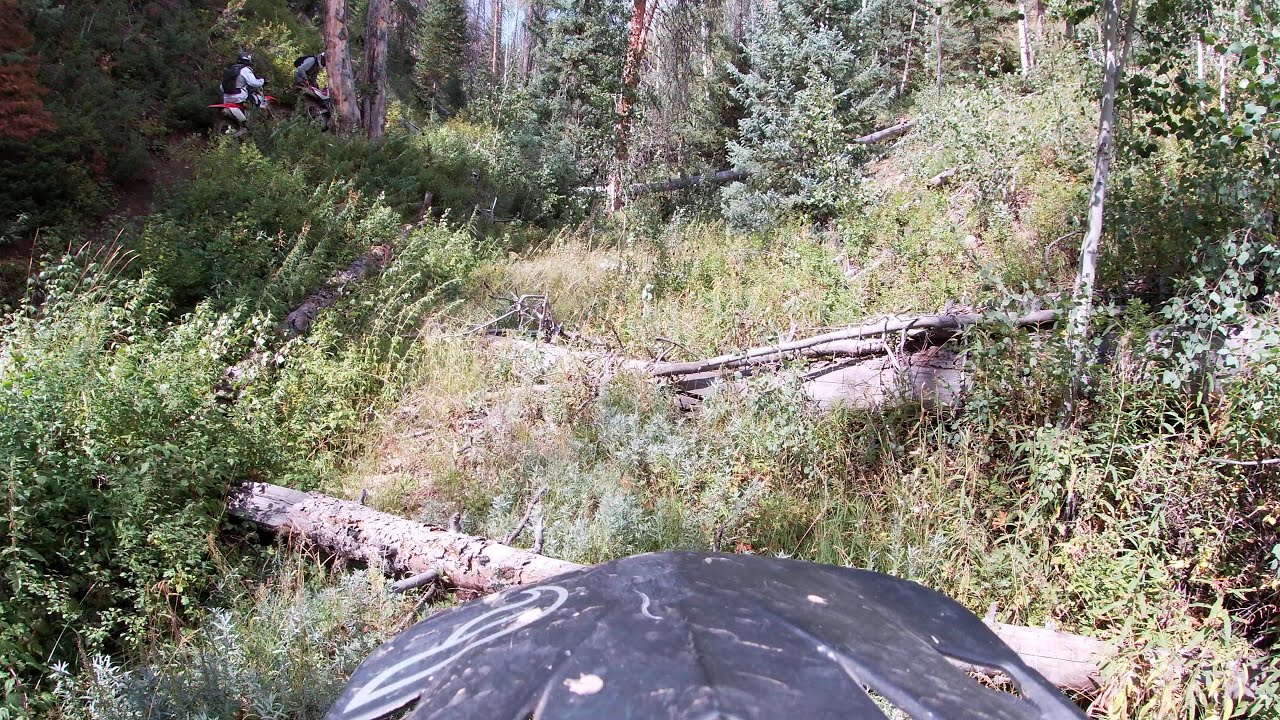In this vibrant daytime scene set in an untouched backcountry area, the image captures two dirt bikers navigating a dense, overgrown forest. The foreground features the black fender of a dirt bike, suggesting a point-of-view shot from a third rider. The forest floor is strewn with fallen logs, thick underbrush, and varying shades of green from the bushes, grass, and towering trees. The bikers, positioned in the upper left of the image, are wearing black helmets and black backpacks. One rider is dressed in a gray shirt while the other sports a white shirt, and both are astride red and white dirt bikes. The sunlight filters through the canopy, casting intricate shadows across the scene, highlighting the wild and uninhabited nature of the terrain. A mysterious black object, possibly a piece of plastic, is centrally located at the bottom of the frame, adding an element of curiosity to the otherwise serene and rugged natural landscape.